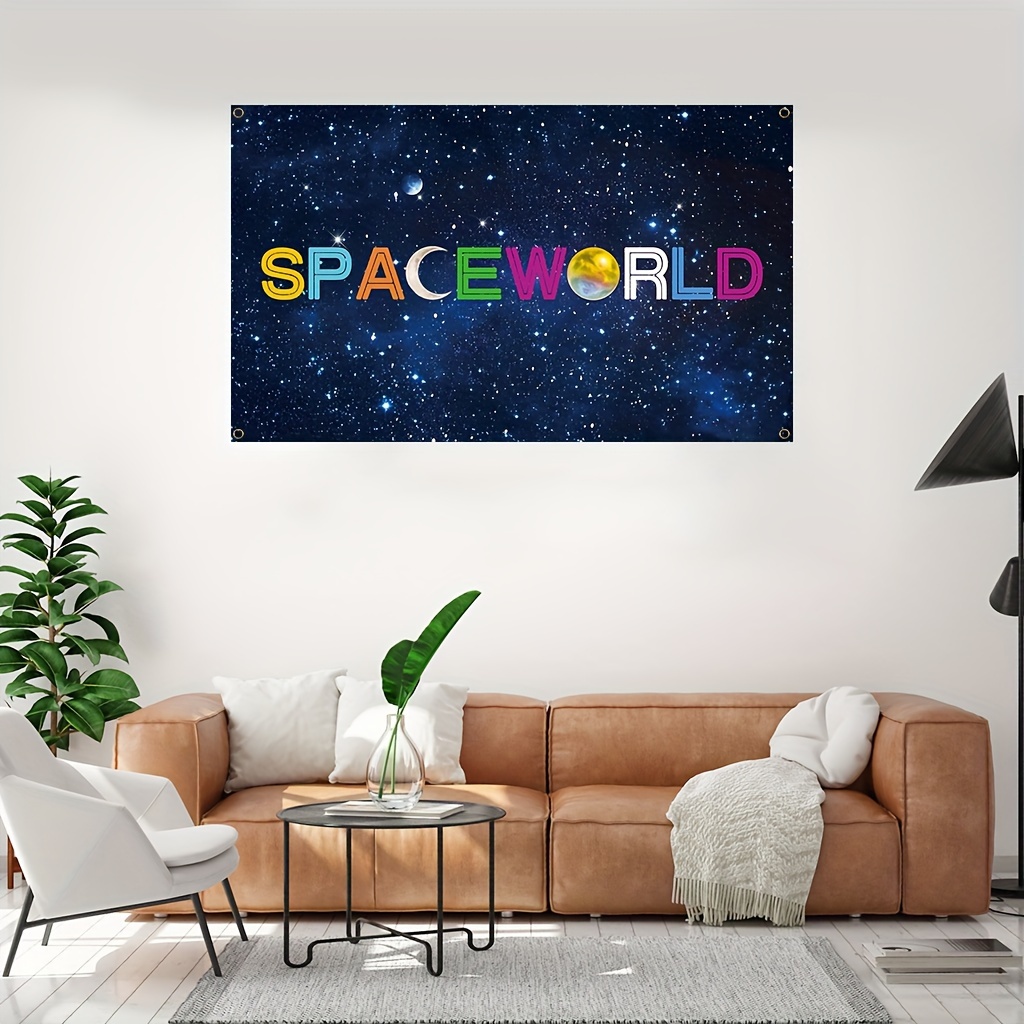The image showcases a cozy living area centered around a vibrant poster hanging on the wall above a brown leather sofa. The poster, titled "Space World," features each letter in a different color—yellow, blue, orange, green, and purple—set against a dark, star-filled space backdrop. The "O" in "World" is depicted as a spherical celestial body resembling Earth, colored mainly in yellow. The living space is accentuated with three white pillows and a white fringed blanket on the sofa. To the left of the sofa, there is a modern white armchair and a tall potted plant. On the right side stands a sleek floor lamp. A round black metal table and a cozy carpet complete the setting, adding to the room's modern and inviting ambiance.